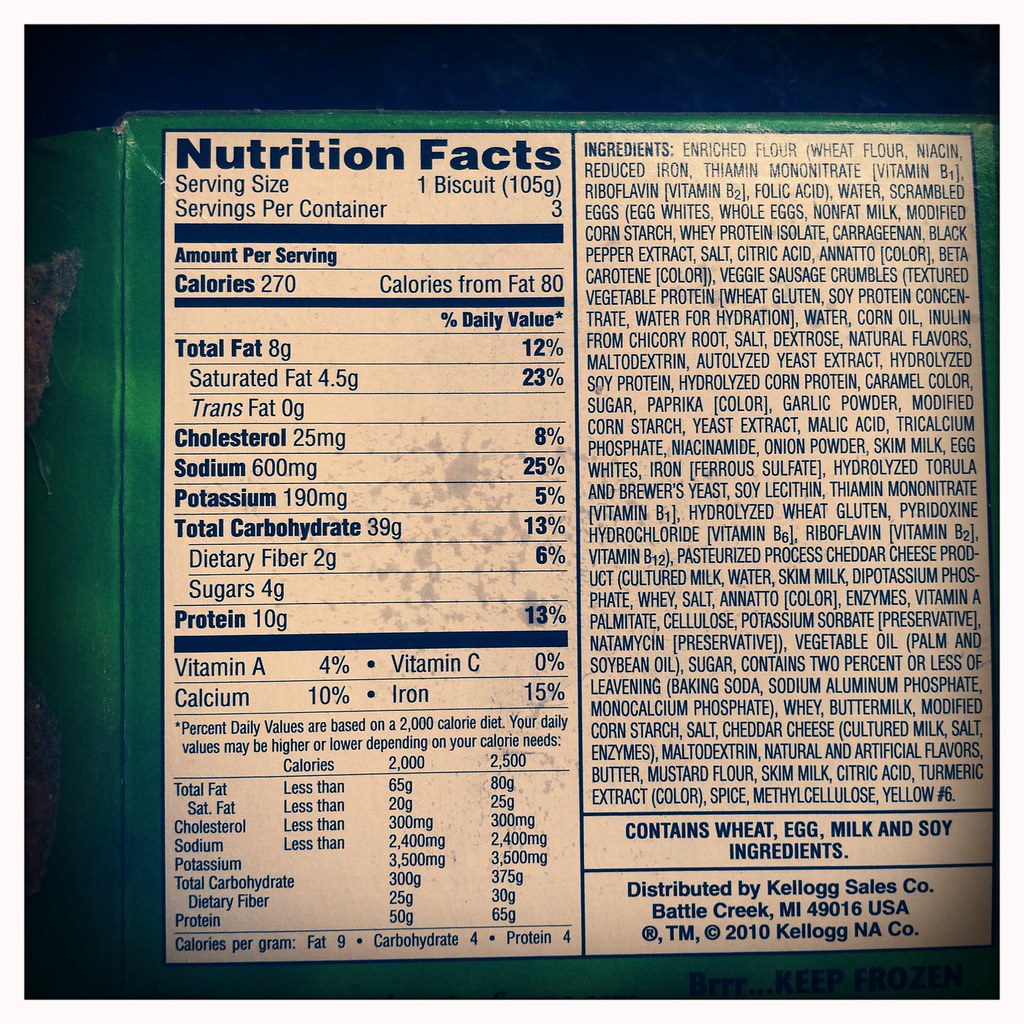This image features the back view of a green food package box, prominently displaying its nutrition label. The label, set on an off-white background with black text, provides detailed nutritional information. The package contains three servings, each serving being one biscuit weighing 105 grams. Key nutritional values are highlighted, including 270 calories per serving, with 80 of those calories derived from fat. The total fat content is listed as 8 grams, cholesterol at 25 milligrams, and sodium at 600 milligrams. Additional nutritional details are also provided on the label, ensuring comprehensive transparency for the consumer.